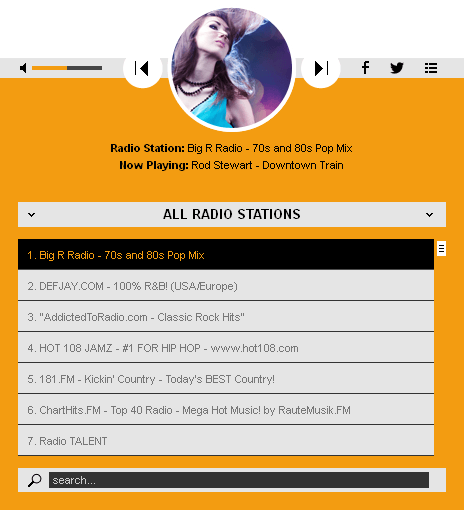The image displays a vibrant interface for a radio station streaming service. In the top-left corner, a sound bar is visible, half-filled in orange, indicating the current volume level. Adjacent to it on the right are rewind and fast-forward buttons.

At the center of the screen, there is a small square with an image of a woman on the left side, set against a vibrant purple background on the right. To the far right of this central section, there are icons for Facebook and Twitter, followed by a horizontal tab menu. The predominant background color of the interface is a warm, goldish-yellow.

Beneath the central image square, small black text reads: "Radio station: Big R Radio 70s and 80s Pop Mix." Directly below, it states: "Now Playing: Rod Stewart - Downtown Train." Another line follows, displaying the text "All Radio Stations" within a light gray rectangle.

Further down, on a black background with gold writing, "Big R Radio 70s and 80s Pop Mix" is prominently displayed. This section lists six radio station options from two through seven:

2. DefJ.com: 100% R&B
3. Addicted2Radio.com: Classic Rock Hits
4. Hot 108 Jams: Number one for Hip-Hop, with a website link
5. 181FM Kicking Country: Today's Best Country
6. Chart Hits FM: Top 40 Radio, mega-hot music by Rot Music FM
7. Radio Talent

Concluding the image at the bottom is a black search bar, allowing users to easily search for specific radio stations or songs.